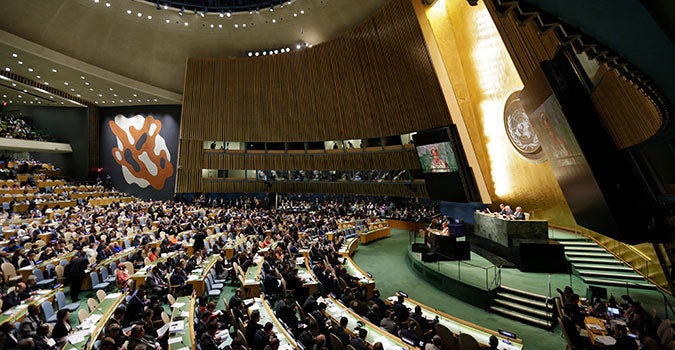The image depicts a massive assembly hall resembling a modern governmental or United Nations meeting. The vast room, possibly accommodating thousands of delegates, features long, curved rows of desks and chairs arranged amphitheatrically, reminiscent of a college classroom. The desks, some with identifying papers, stretch from the front to the back of the hall, filled with representatives from various countries or regions, all engaged in discussions.

Centrally, there is a distinctive green-floored area with a multi-tiered platform. The highest platform holds a large bench akin to a judicial setting, where three key figures are seated, likely moderating the proceedings. To the side, additional tables with computer monitors and a vivid yellowish backdrop bearing a round governmental emblem are visible, lending an official atmosphere.

Overhead, large TV screens focus on the current speaker, ensuring visibility for all attendees. The hall's backdrop features a yellow wall emblazoned with a globe-like artwork, underlining the international or global theme. The ambient light brightens the room, highlighting the hall's detailed architecture, including portions of orange, blue, gray, and white hues that add to the modern aesthetic.